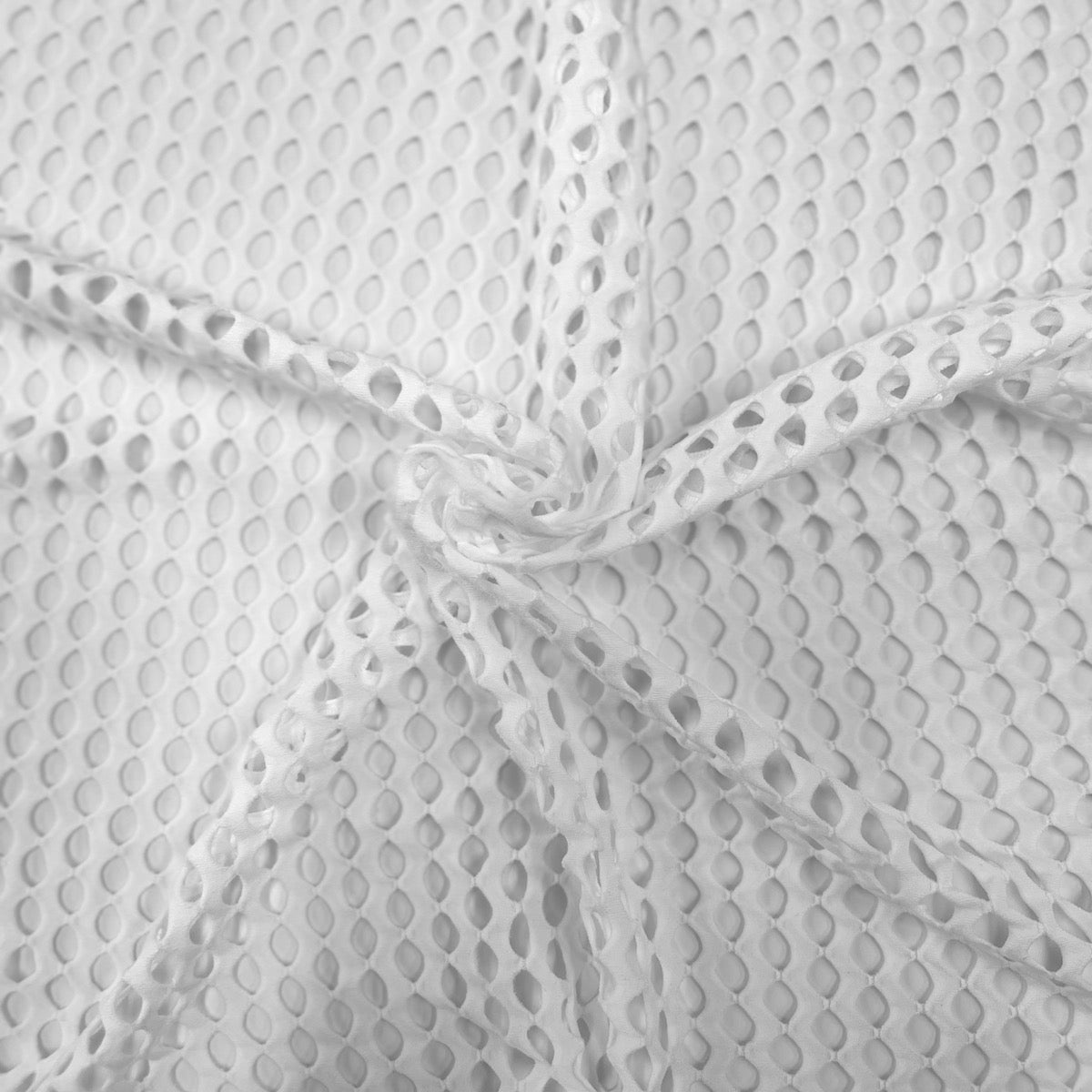This color photograph, taken in a square format, features a piece of white eyelet fabric that is laid flat against a white background. The fabric has a distinctive netting appearance with multiple rows of cylindrical cut-out shapes that allow the background to show through, creating a textured look. The focal point of the image is a central knot where the fabric has been twisted, generating radiating folds that form a star-like or floral pattern. The twisting manipulation pulls the fabric into distinct lumps and folds that spread outward, creating a dynamic and intricate design that gives the material a three-dimensional quality. Photographed in the style of representational realism, the image captures the detailed texture and structure of the fabric, highlighting its delicate and uniform pattern.